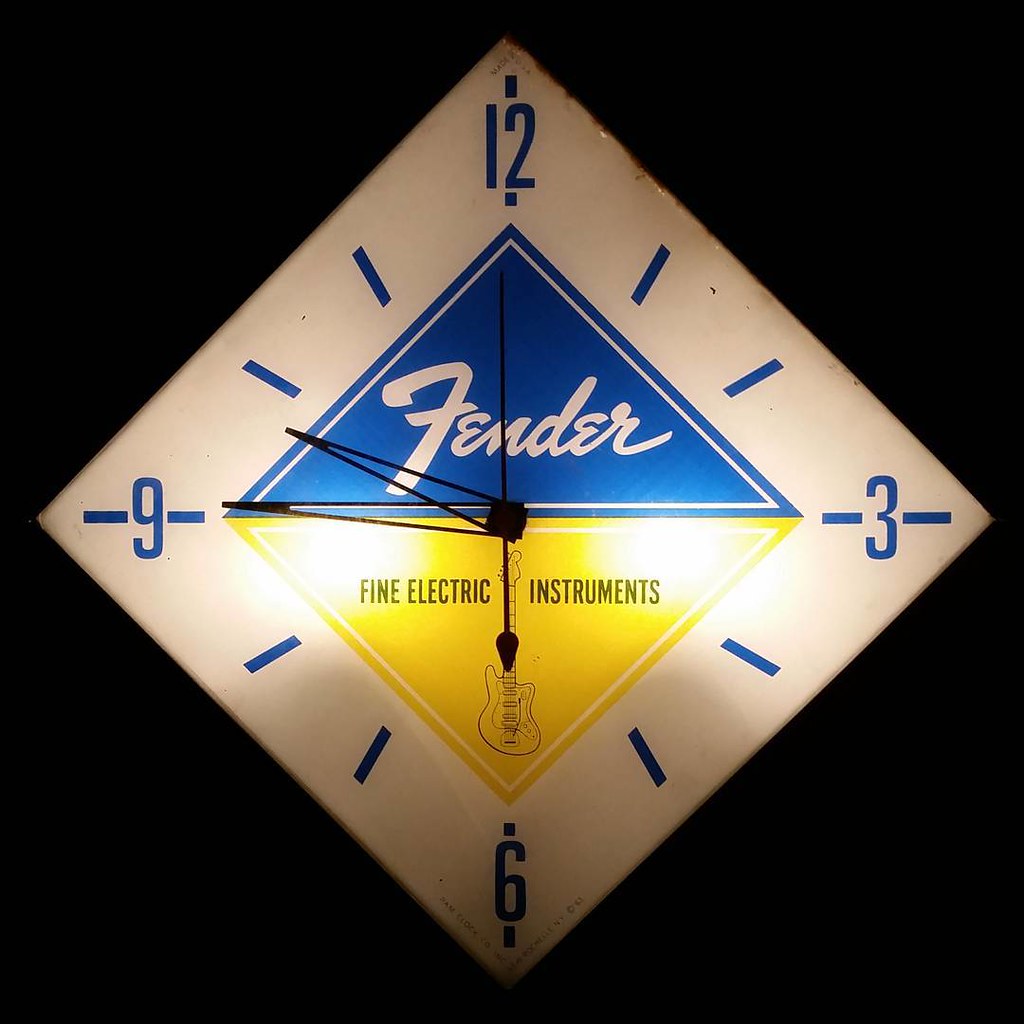This striking photo features a unique clock set against an almost entirely black background, emphasizing its standout design. The clock is diamond-shaped, resembling a perfect square rotated 45 degrees. Its minimalist face showcases the numbers 12, 3, 6, and 9 in a vibrant blue color, while the other hour markers are indicated by longer dashes without numerical labels. At the very center, an additional diamond shape is divided into two parts: the top half forming a blue triangle emblazoned with the "Fender" logo in crisp white letters, and the bottom half appearing in yellow with the text "Electric Instruments," accompanied by an outline illustration of a guitar in a darker hue, likely black.

The clock is further adorned with delicately thin, wire-like triangular hands that point to the time, which is accurately depicted as 9:45. Present also is a seconds hand, maintaining the clock's cohesive design aesthetic. The simplicity of the clock's face, combined with the sharp contrast against the dark background, creates a visually captivating and elegant timepiece.